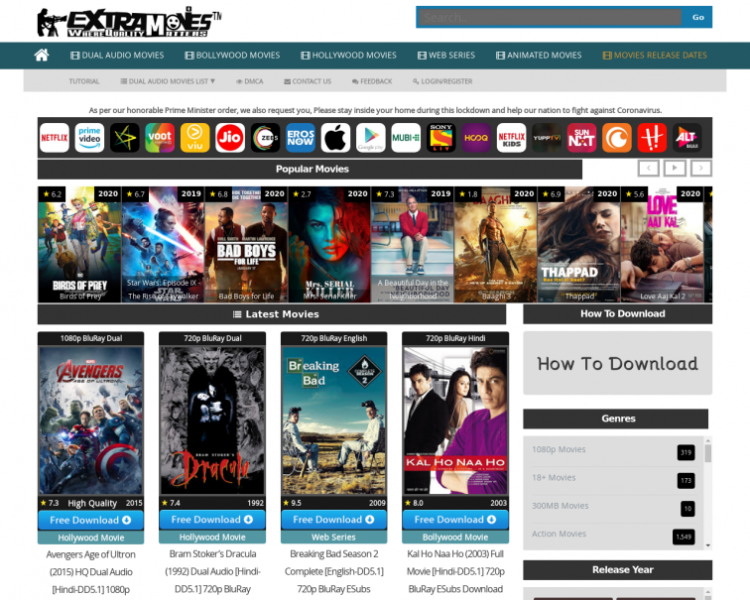A screenshot from a website showcasing a variety of movie options. In the top left corner, a black-and-white logo reads "Extra Movies: Where Quality Matters." Adjacent to this, a blue-bordered search bar with an empty gray rectangle invites user input, with the word "Go" in white on a blue button to the right. Beneath the search bar, a long horizontal navigation bar includes categories and a small white home button. Another light gray horizontal bar below it lists additional categories.

Further down, a section filled with colorful widgets from various apps and platforms like Netflix and Prime Video cascades across the screen. Below this, an extensive array of movie options is presented with their covers prominently displayed, and release dates indicated in small black boxes located in the top right corners of each movie image. Featured titles include "Birds of Prey," "Star Wars Episode," and "Bad Boys for Life." Additional movies listed at the bottom encompass "Avengers," "Dracula," "Breaking Bad," and "Kal Ho Naa Ho." 

A sidebar on the right side contains a gray rectangular box with instructions on "How to Download," followed by a section labeled "Genres." The screenshot captures a well-organized, comprehensive interface tailored for movie enthusiasts.